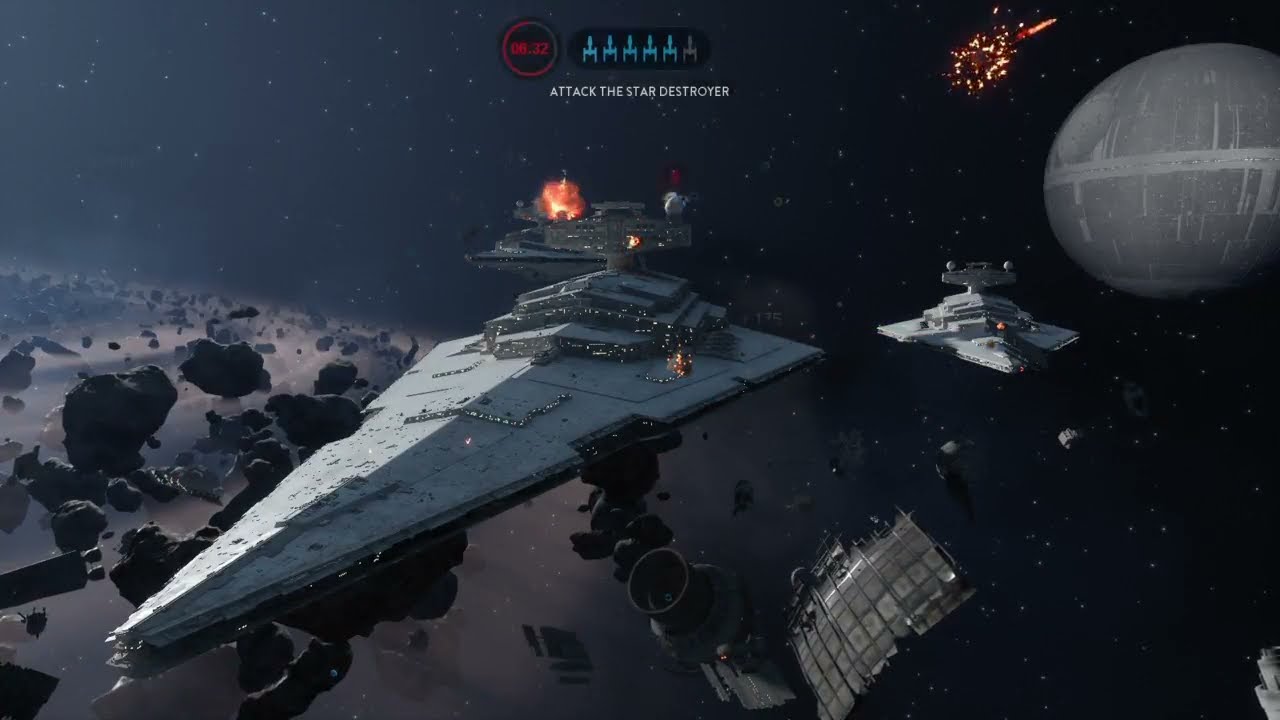This image is a detailed screenshot from a Star Wars-themed video game, set in an outer space environment filled with stars scattered across a black sky. Dominating the image, a large triangular Star Destroyer floats centrally, with intricate details including illuminated towers and various lights indicating inhabited areas. To the right, a smaller spaceship resembling a bomber plane is visible, while in the backdrop, another round spaceship appears to be exploding, emitting flames. Surrounding the scene are numerous asteroids and meteors forming an asteroid belt, enhancing the sense of a chaotic space battle. In the upper right corner, the Death Star looms with gray tones, adding to the Star Wars ambiance. Towards the bottom, space debris, likely remnants of destroyed ships, is discernible. The upper part of the screen displays a mission objective that reads "Attack the Star Destroyer," accompanied by a red circular timer, signaling a time-sensitive task. Additionally, the top of the screen features a mission status box showing icons of six ships, with five in blue and one grayed out, indicating either destroyed ships or lost lives in this intense skirmish.